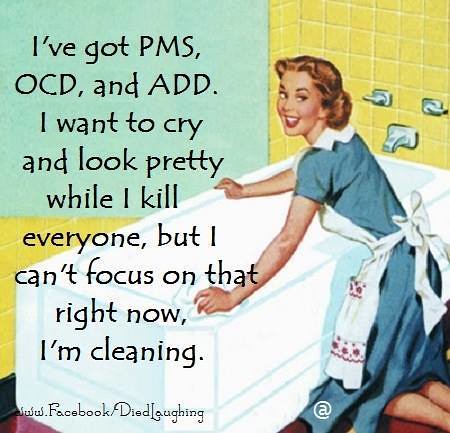The image appears to be a vintage-style advertisement reminiscent of the 1950s, blending old-school aesthetics with modern humor. It features a woman dressed in a blue house dress and white apron, complete with coiffed hair and red lipstick, kneeling in front of a white bathtub with stainless steel spouts and two levers. The background showcases yellow tiles surrounding the bathtub. Overlaying the image, in the top left corner, is a blue, rectangular background with bold black text that humorously reads: "I've got PMS, OCD, and ADD. I want to cry and look pretty while I kill everyone, but I can't focus on that right now. I'm cleaning." At the bottom left of the image, there's a website link, "www.facebook.com/diedlaughing," along with a small copyright mark in white at the center bottom of the page.